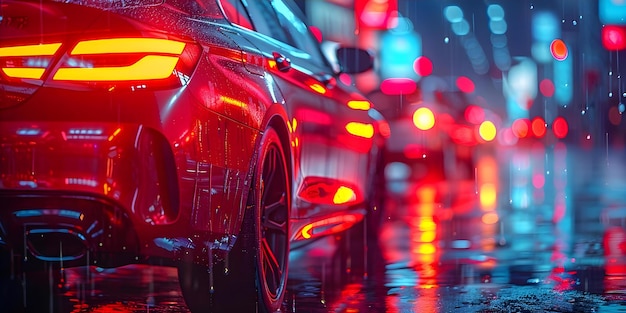A photograph captures a nighttime street scene on a rainy day. Water droplets splashed onto the camera lens add to the ambiance, reflecting light in a way that obscures the whole right side of the image. The road surface at the bottom of the image is wet and highly reflective, enhancing the shimmery effect of the setting. Dominating the left side of the image is a sleek sports car, potentially red, with its brake lights illuminated. The car has bright yellow lights and dual exhausts, and its exterior is covered in rain droplets, adding to the overall shimmering look. The car occupies the left-hand portion of the image and its presence is magnified by the reflections of red and yellow neon lights from the surrounding cityscape. The background is blurred but suggests a bustling, metropolitan environment with hints of other cars and distant lights, predominantly in shades of red, blue, and yellow. The wet pavement and the neon reflections contribute to the image's vibrant, almost cinematic quality.